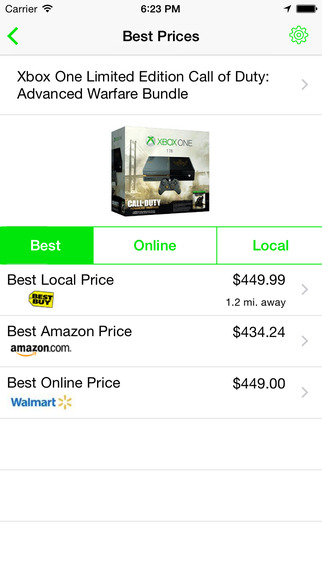The image is a screenshot from a smartphone showcasing a price comparison for the "Xbox One Limited Edition Call of Duty: Advanced Warfare Bundle." The screen is divided into sections, each dedicated to different purchasing options. At the top, prominent text reads "Best Prices." Below that, the screen is divided by faint gray lines into three sections labeled "Best," "Online," and "Local."

In the "Best Local Price" section, the price is listed as $449.99. The location is specified as Best Buy, situated 1.2 miles away. In the "Best Amazon Price" section, the price is $434.24 from Amazon.com. The "Best Online Price" section shows the price as $449.00 at Walmart.

Additional details at the top of the screen show a fully charged battery icon in black, the word "Carrier," a Wi-Fi signal icon, the time "6:23 p.m.," a gear icon possibly for settings, and a back button with an arrow pointing back.